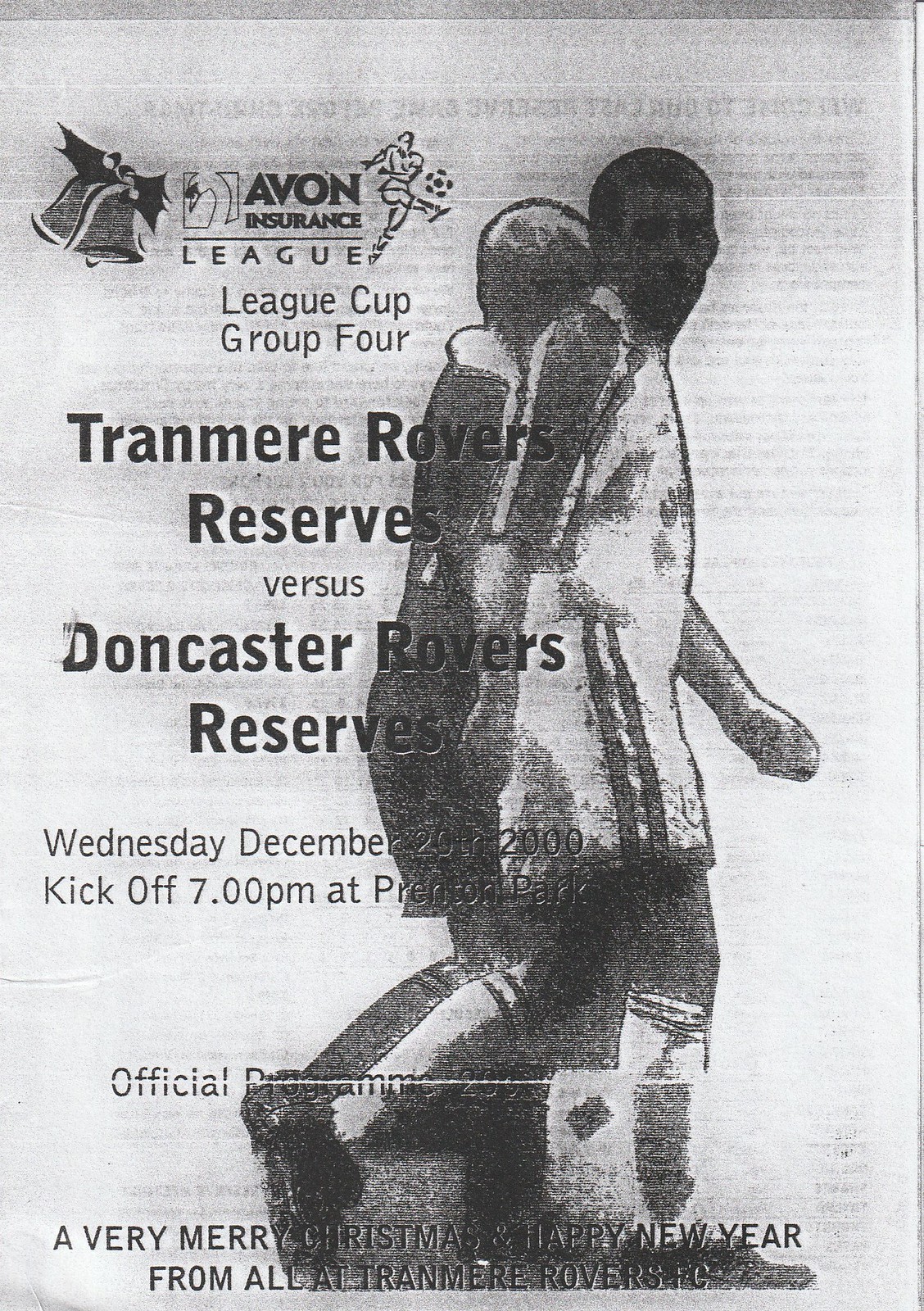A black and white poster features a prominent heading sponsored by Avon Insurance at the top left, signifying the League Cup Group 4 match between Tranmere Rovers Reserves and Doncaster Rovers Reserves. The match details state a kickoff on Wednesday, December 20th, 2000, at 7 p.m., at Plankton Park. The image showcases a pixelated, grainy drawing of two soccer players walking in stride, one in a lighter uniform and the other in a darker one. Adding to the festive spirit, the bottom of the poster conveys a warm message: "A very Merry Christmas and Happy New Year from all at Tranmere Rovers FC." Additionally, Christmas bells adorn the left side of the image to complement the holiday greeting.